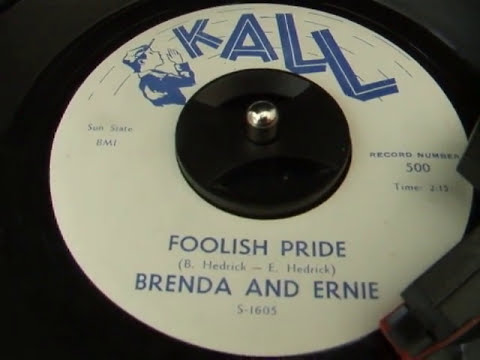This detailed caption combines the key elements from all three descriptions to create a comprehensive and coherent narrative of the image:

The image displays the label of a vintage 45 RPM vinyl record, which traditionally features a large central hole, clearly visible here with a black spindle and a small silver knob typical of record players. The photograph is framed in a small square format, with the corners showing a dark black background that blends into the equally dark base beneath the record. 

Dominating the center of the record is a white circular label. At the top, prominent in large blue uppercase letters, is the logo K-A-L-L. Accompanying the logo is an illustration of a boy, possibly a Boy Scout, who appears to be shouting or calling out, with his hand raised near his face and an action line accentuating the dynamic. Just beneath the logo, the label details "Sunstate BMI" on the left side and "Record number 500" on the right, along with a playing time marked as "2:15."

The title of the song, "Foolish Pride," is also printed in blue capital letters, followed by the credits to B. Hedrick and E. Hedrick, identifying Brenda and Ernie as the performers. The label further specifies the catalog number S-1605 at the bottom, all in a matching blue font.